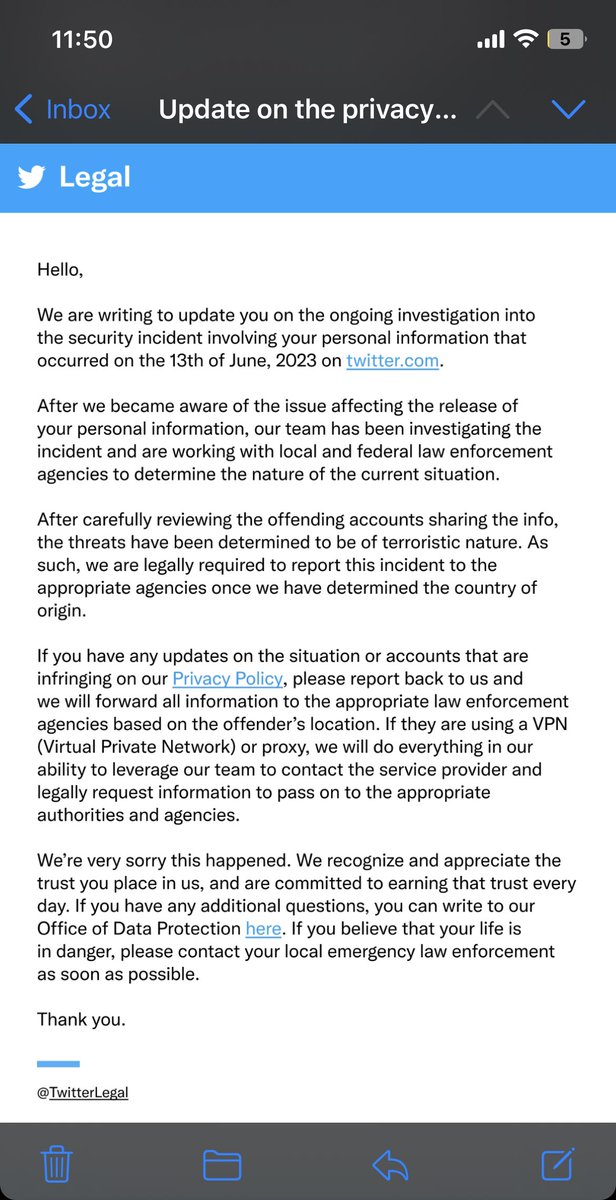Screenshot of a phone taken at 11:50 AM, showing full data bars, a Wi-Fi symbol, and a battery icon at the top right. The screen displays a message from Twitter within a white background. The message, titled "Legal," is set against a blue header with a white bird logo. It details an ongoing investigation into a security incident involving the recipient's personal information that occurred on June 13, 2023. The message apologizes for the breach and provides updates on efforts to resolve the issue. At the bottom of the screen, the interface includes icons for a trash can folder, a back arrow, and a square with a pencil. The top and bottom of the screen have gray backgrounds.